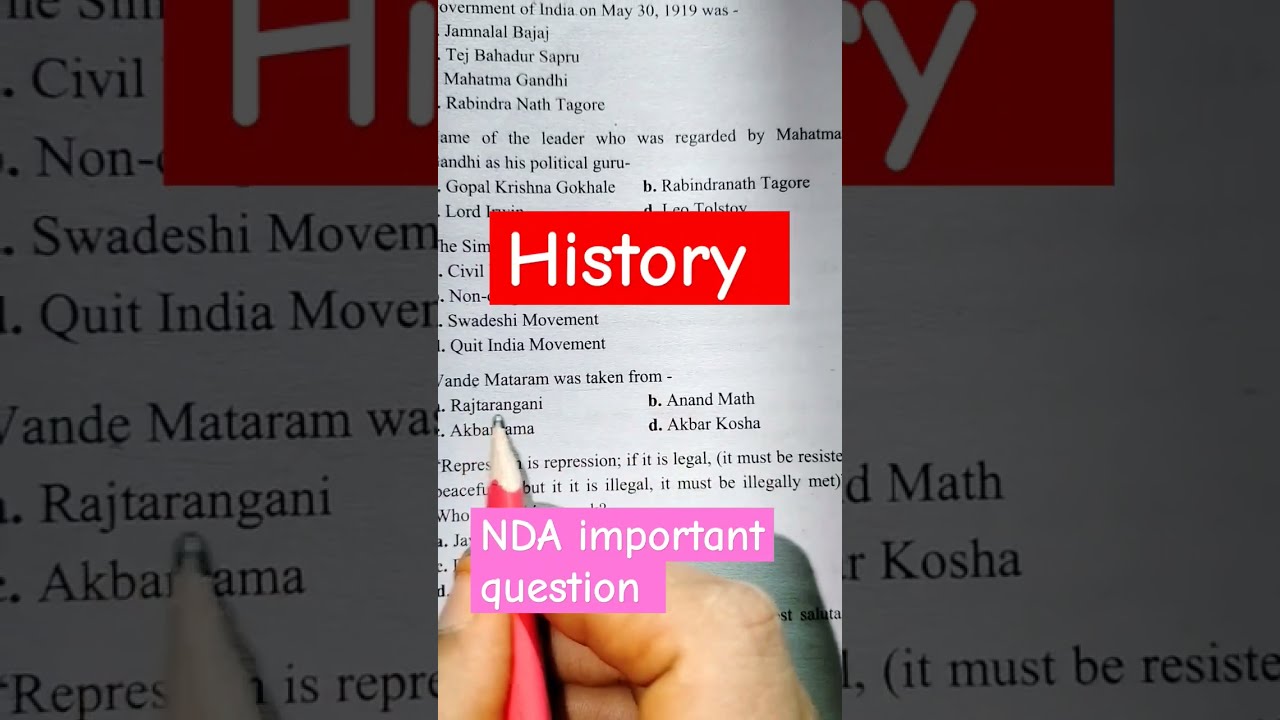The image depicts a section from a textbook or multiple-choice test, showcasing various questions and answers. Dominating the center is a red rectangular text box with "history" written in white Comic Sans-style font, and beneath it, a pink text box that reads "NDA, important question" in the same font. Both the left and right thirds of the image are dimmer and appear to be zoomed-in sections of the center image. In the foreground, the focus is on a person’s right hand, specifically the thumb and fingers, holding a red wooden pencil, which appears slightly dull at the tip. The pencil is pointed towards the word "Rajatangani." The sheet of paper is white, with questions and answers formatted in a multiple-choice style, marked with letters A, B, C, and D. This image seems like it might have been captured for an Instagram story or TikTok reel, based on the aspect ratio suggesting a smartphone screen.